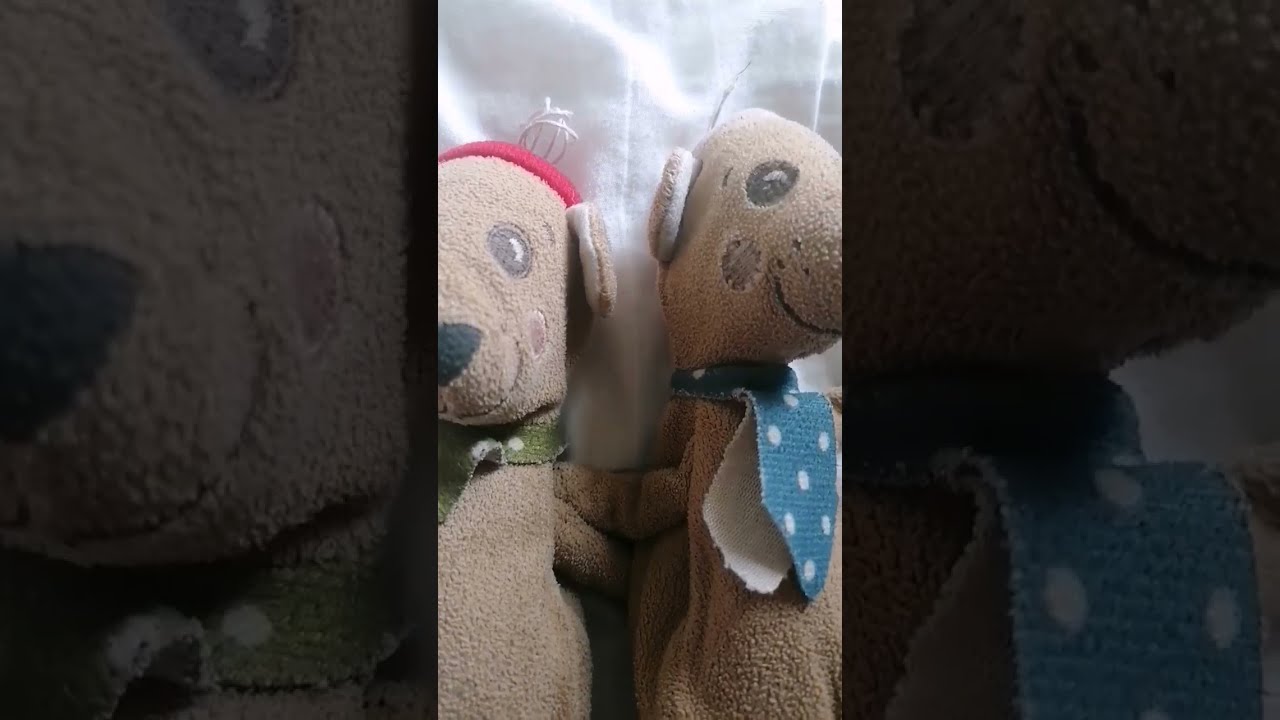This is a horizontal rectangular photograph divided into three panels. The center panel is a close-up of two cartoony stuffed dogs lying side by side on a white cloth, with arms stretched out and touching each other's backs. Both dogs have drawn or colored-in brown circular eyes, black noses, and smiling mouths. The dog on the left sports a red beanie and a green polka-dotted scarf, while the dog on the right wears a blue polka-dotted scarf. Their brown fur and similar features suggest they are twin-like in appearance. The top of the center panel shows a light source coming from the ceiling. 

The left panel of the photograph is a shaded close-up of the dog on the left, highlighting its red beanie and green scarf. The right panel is another shaded close-up but focuses more on the blue and white polka-dotted scarf of the dog on the right. Both side panels are darker in contrast to the central image, emphasizing the stuffed toys' accessories and features.